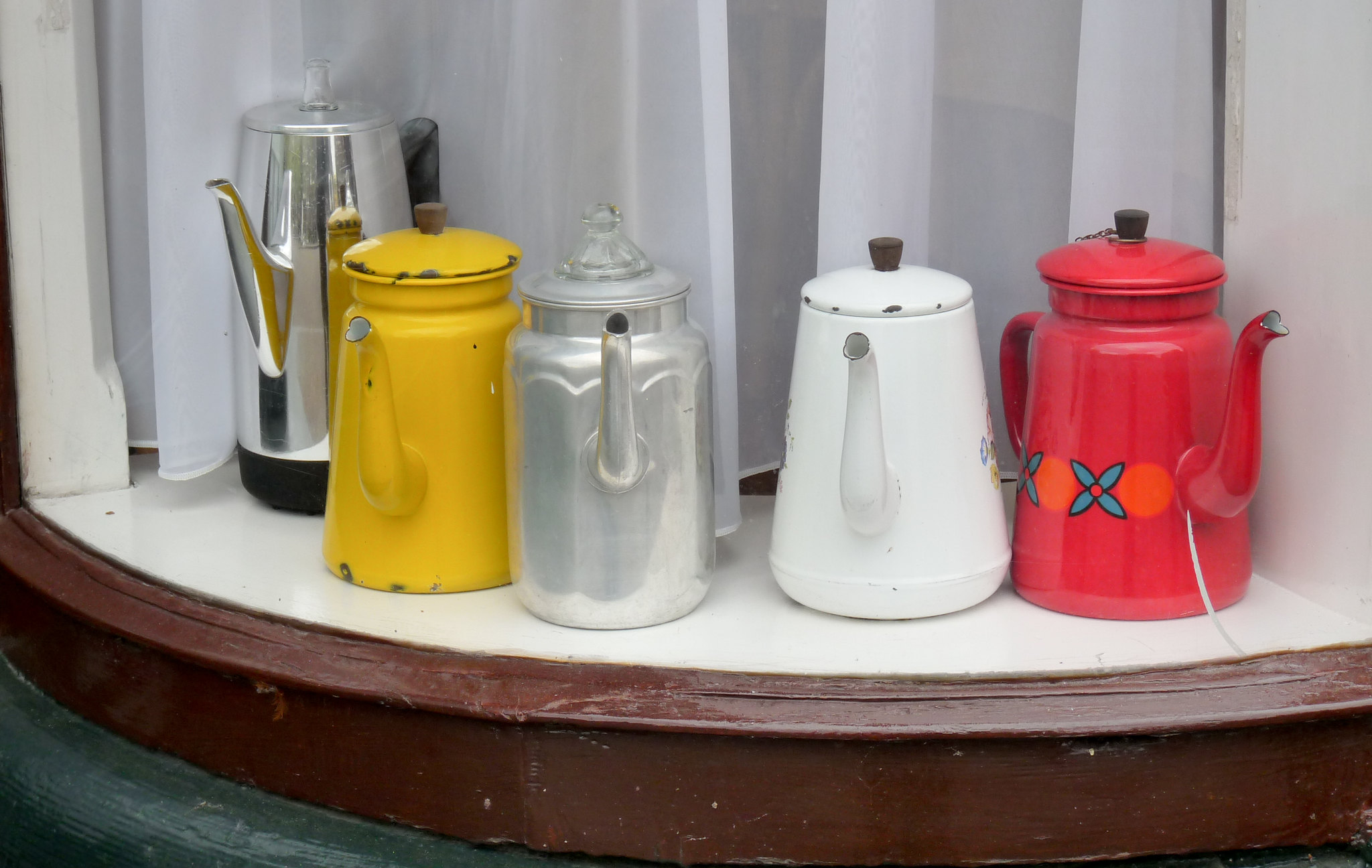This detailed scene captures a collection of five distinct teapots arranged on a white-painted windowsill, partially covered by a sheer white curtain. The wooden trim of the shelf adds a rustic touch, while the wall behind, described as a dark greenish-black hue, contrasts with the vibrant colors of the teapots. From left to right, the first teapot is a modern, tall, silver one with a chrome finish and a black bottom. Next is an older, well-used vibrant yellow teapot with a slightly rusty top and a small wooden handle. To its right is a thicker, less shiny metal teapot, likely aluminum, with a silver finish. Following this, there is a white teapot adorned with small white dots on the lid and a black handle, exhibiting signs of rust. The final teapot is a striking fuchsia pink, featuring blue flower designs and additional orange circles, with a pristine appearance as though it were recently purchased, its red handle and white interior further emphasizing its vivid presentation.